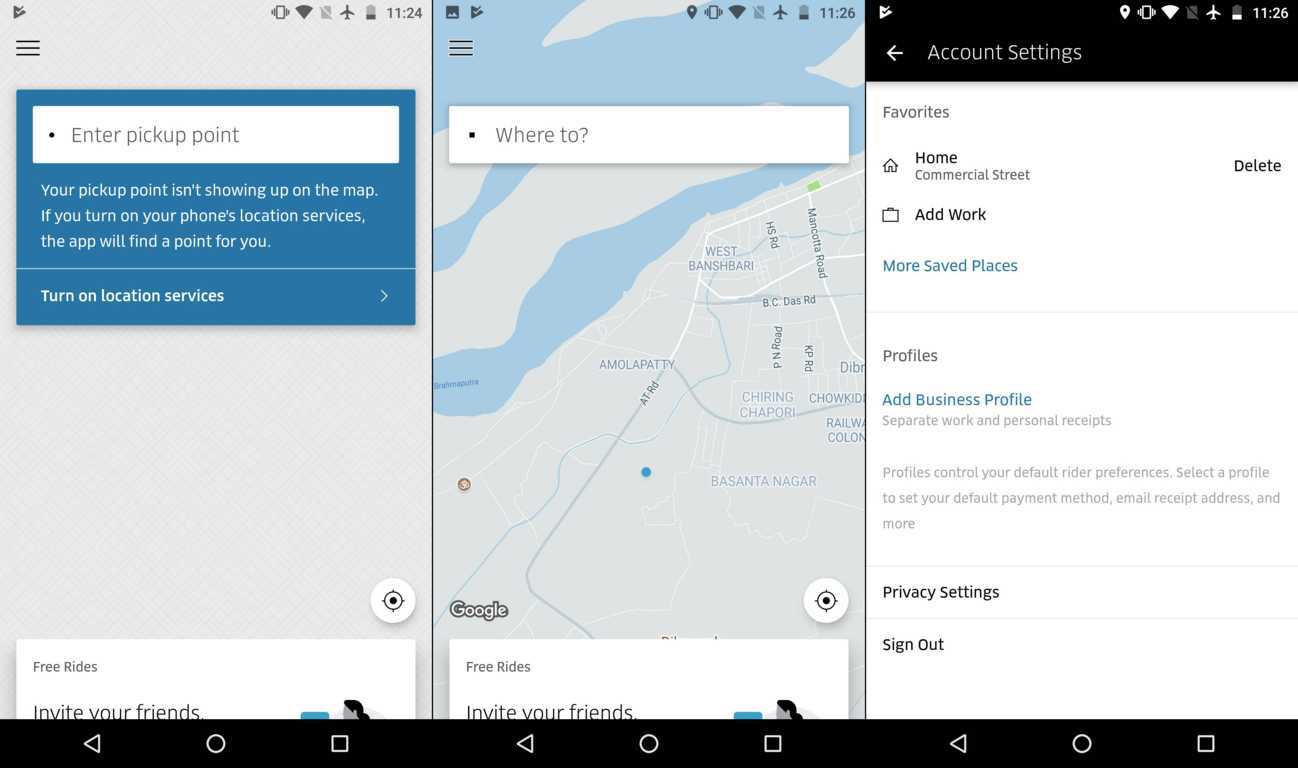This series of three side-by-side smartphone screenshots provides an in-depth look at different functionalities within a mobile application. 

The first screenshot on the left showcases the 'Pickup Point' entry screen. A search bar at the top allows users to input their desired pickup location, accompanied by a helpful tip below which suggests enabling the phone's location services for more accurate pin-pointing. There's a clickable option to turn on location services immediately.

The central screenshot presents a detailed map brimming with rivers and lakes, illustrating a specific geographic area. A prominent search bar labeled "Where to?" invites users to set their destination.

The third screenshot on the right displays the 'Account Settings' page. At the top are 'Favorites,' listing saved locations like 'Home' and 'Commercial Street,' complete with options to either delete these entries or add new ones. A 'More Saved Places' link is available for further customization. Below this, there's a 'Profile' section for adding a business profile, which appears to be empty. The bottom portion contains 'Privacy Settings' and an option to 'Sign Out.'

All three screenshots include the familiar phone menu bars at the top and bottom, providing a cohesive and user-friendly experience.